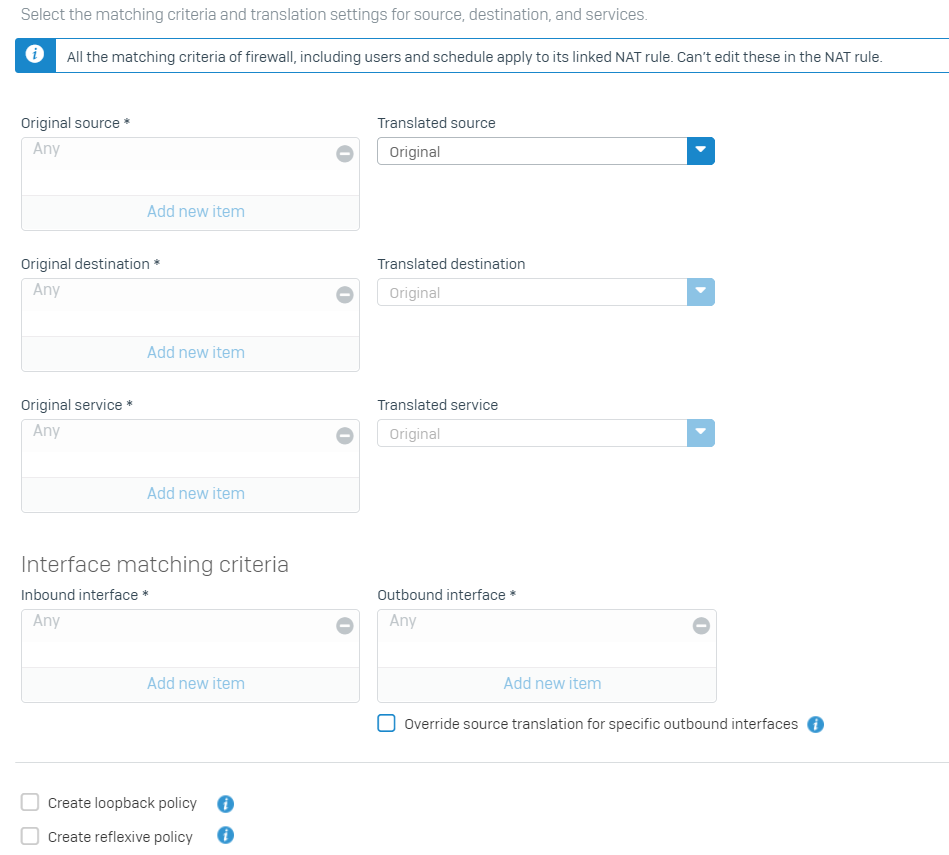Image Caption: 

At the top, the window displays a gray header with the text: "Select the matching criteria and translation settings for Source, Destination, and Services."

Beneath this header, a noteworthy section includes a small blue square with a white "i" icon, and the adjacent text reads: "All the matching criteria of Firewall, including users and schedule, apply to its linked NAT rule. You can't edit these in the NAT rule."

The left-hand side features a series of gray input boxes labeled as follows:
1. "Original Source *"
2. "Original Destination *"
3. "Original Service *"
4. "Inbound Interface *" (preceded by the heading "Interface Matching Criteria")

On the right-hand side, corresponding drop-down boxes read:
1. "Translated Source" with "Original" selected.
2. "Translated Destination" with "Original" selected.
3. "Translated Service" with "Original" selected.
4. "Outbound Interface *" 

Below these, there's an option within a blue box: "Override source translation for specific outbound interfaces."

A gray horizontal line separates this section, followed by two additional options represented by small checkboxes:
1. "Create loopback policy"
2. "Create reflexive policy"